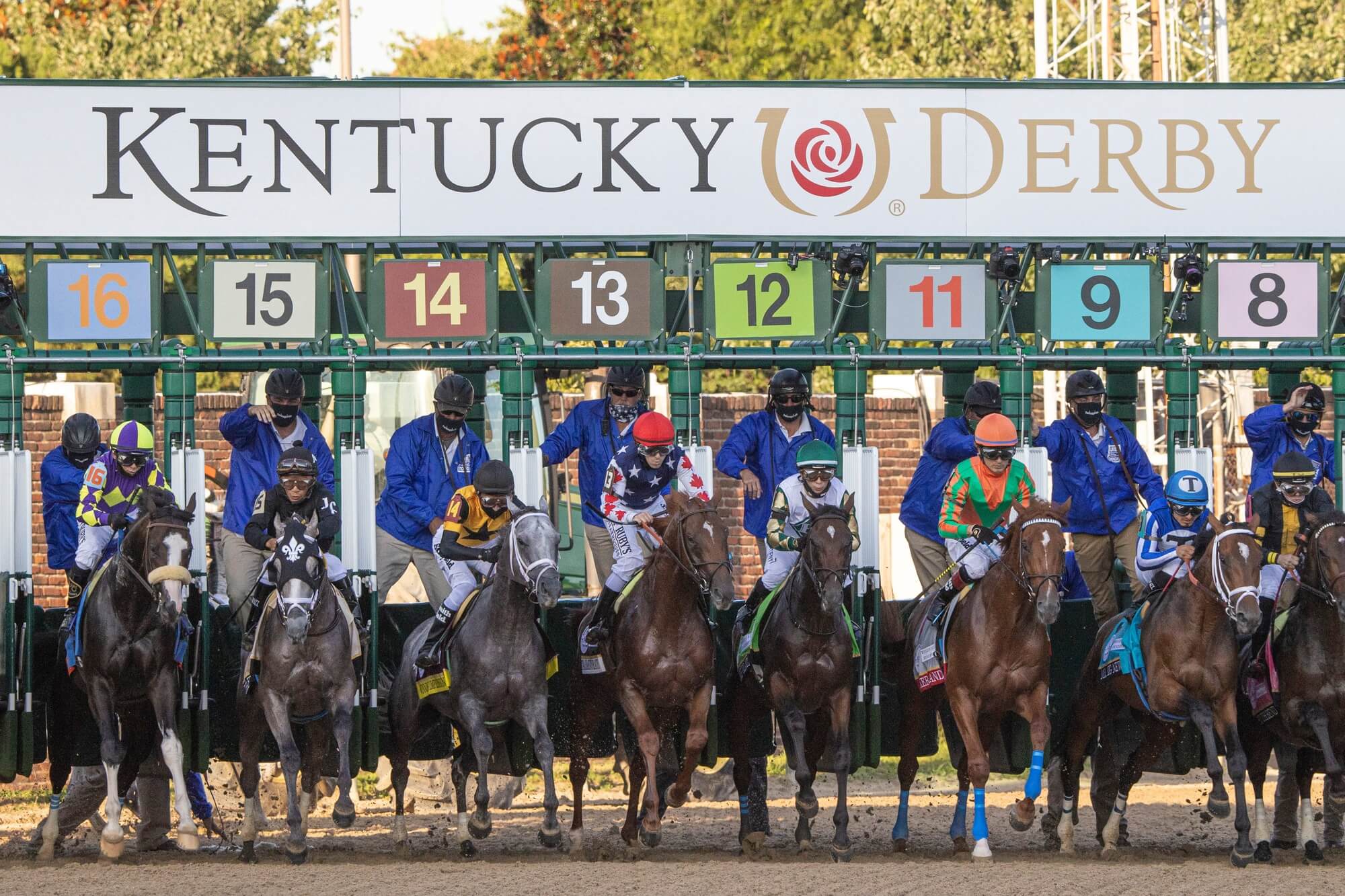The image captures the dramatic start of the Kentucky Derby, a horizontal rectangular photograph showing horses bursting out of the green metal starting gates, which are numbered from 8 to 16. Above the gates, a large white banner prominently reads "Kentucky Derby" with "Kentucky" in black and "Derby" in gold, separated by a small logo featuring a horseshoe and a rose. Each horse is a different color, with some being black, gray, or brown, and many bearing distinct white markings on their foreheads. The jockeys, sporting various brightly colored uniforms that match their helmets, are all poised for the race. Behind each jockey stands an attendant in a blue jacket, wearing a helmet and black face mask, readying the horses for their swift start. The ground beneath the horses is a light brown dirt, capturing the energy and anticipation of the race’s commencement as the number 9 horse leads the charge. The tops of lush green trees are visible in the background above the banner.